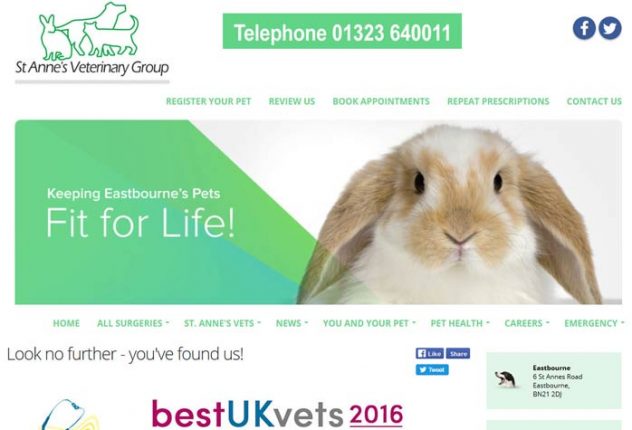In the upper left corner of the image, the signage reads "St. Anne's Veterinary Group." Centrally positioned is a contact number, "Telephone: 01323 640011," flanked by Facebook and Twitter icons on the right. Across the middle of the image, there is a navigation menu featuring options such as "Register Your Pet," "View Us," "Book Appointments," "Repeat Prescriptions," and "Contact Us." Prominently displayed in the center is a photograph of a bunny with its ears down, showcasing a brown and white fur pattern.

On the left side of the image, text reads, "Keeping Eastbourne's pets fit for life," with the word "Eastbourne" highlighted. Below this, an additional navigation menu includes dropdown options for "Home," "All Surgeries," "St. Anne's Vets," "News," "You and Your Pet," "Pet Health," "Careers," and "Emergency." Further down, a message on the left states, "Look No Further, You've Found Us," accompanied by Facebook Share and Twitter icons. On the right, an address is partially visible: "Eastbourne, 5 East Annette's Road, Eastbourne BNQ12DJ" (the exact postcode is indistinct due to low resolution).

Toward the bottom middle, a badge declares "Best UK Vets 2016." The overall color scheme of the image includes shades of green, gray, white, blue, brown, white, and a hint of pinkish purple.